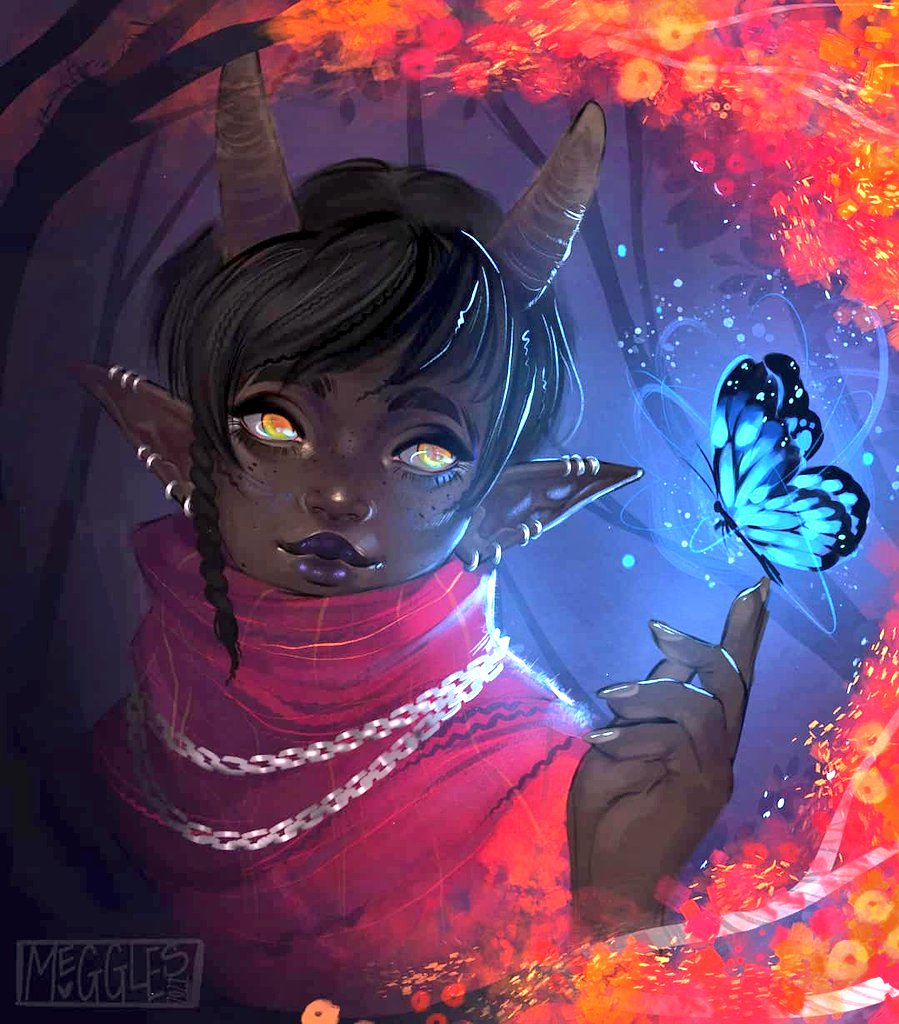This artwork, crafted by the artist Meggles (signature in the bottom left corner), depicts an unusual and captivating fairy-like figure. The fairy has striking black hair, styled with a braid on the right side, and adorned with goat-like horns protruding from her head. Her pointed, elfin ears are decorated with silver rings, enhancing her mystical appearance. The fairy’s eyes are mesmerizing gold, and her lips are painted a deep purple.

She dons a pink turtleneck shirt, accessorized with two silver chain necklaces. Her skin has a rich, brown tone. Her right hand is raised with her index finger extended, gently supporting a beautiful blue and black butterfly, caught mid-flap, as indicated by the dynamic brush strokes around it. 

The background features soft oranges, ambers, and yellows, with flowing red and orange flowers cascading from the top right to the bottom right. The subtly painted trees add depth and a dreamy quality to the setting, which is primarily awash with purple hues and orange highlights.